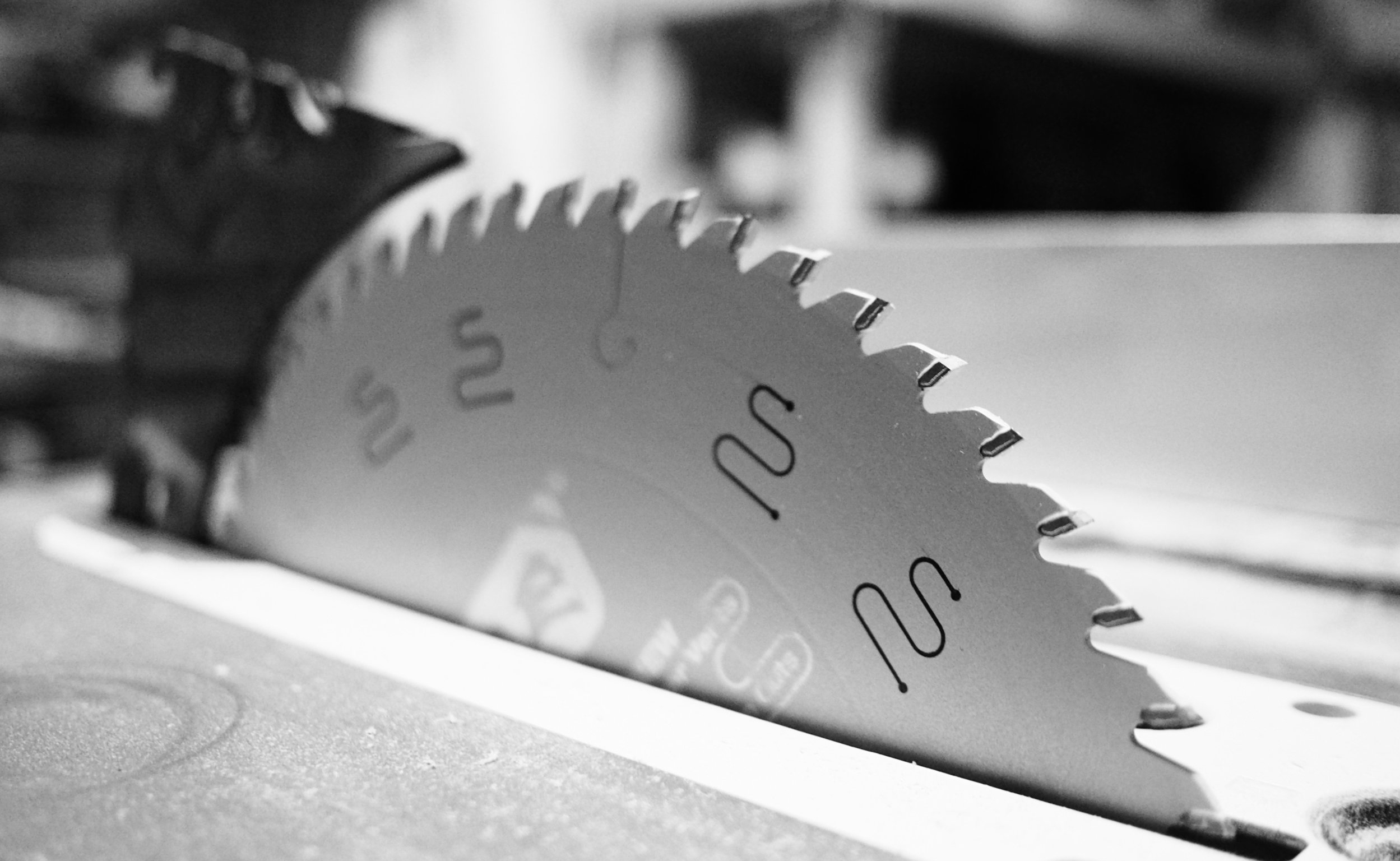This detailed, black and white close-up image showcases a pristine circular saw blade emerging from a stationary table saw. The blade is the clear focal point of the photo, with its sharp, serrated edges and intricate snaked pattern cut through about halfway down, adorned by four sets of squiggly lines and a central hook design. Despite its brand-new appearance, indicated by the crisp and unread white writing on its surface, the surrounding saw table tells a different story with visible fine dust and sawdust scattered across its silver surface. The background fades into obscurity, featuring blurred metallic fixtures and what appears to be a factory setting or reflection, adding an industrial ambiance without drawing attention away from the detailed saw blade. The black plastic guard at the back of the blade is indistinct, reinforcing the emphasis on the sharp, immaculate blade that commands the scene.